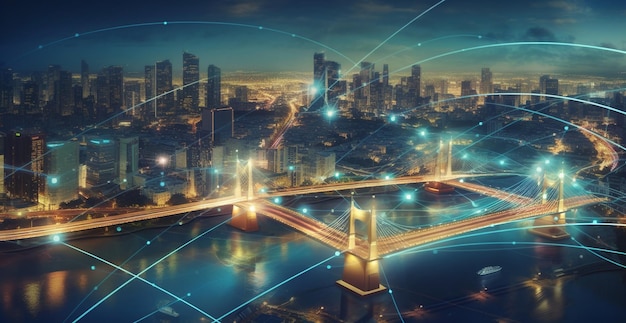This piece of digital artwork intricately depicts a bustling cityscape at night. The foreground features a prominently illuminated suspension bridge arching over a very clear body of water, reflecting the bridge and city lights in its serene surface. The bridge exhibits a distinctive design, possibly including a square element, which seems to manage traffic flow between the city's sections flanking the river, potentially leading into an ocean. The river is tranquil, dotted with a few boats, enhancing the serene yet lively atmosphere.

In the background, a densely developed skyline of towering skyscrapers stretches across the horizon, their many windows emitting a subdued yellow glow, punctuating the night with a quiet vibrancy. Behind these buildings, brightly lit highways weave through the urban jungle, adding depth and complexity to the cityscape.

The sky itself is a gradient of dark blue-gray to almost black, adorned with artistic strings and points of light that resemble stylized stars, lending the scene a dreamlike quality. This ethereal effect is further emphasized by the entire image's subtle blue tint, giving it a cohesive, almost surreal aesthetic. Despite the detailed and busy urban environment, the picture maintains a calm, almost otherworldly beauty, with no visible cars or people to clutter the serene nocturnal vista.